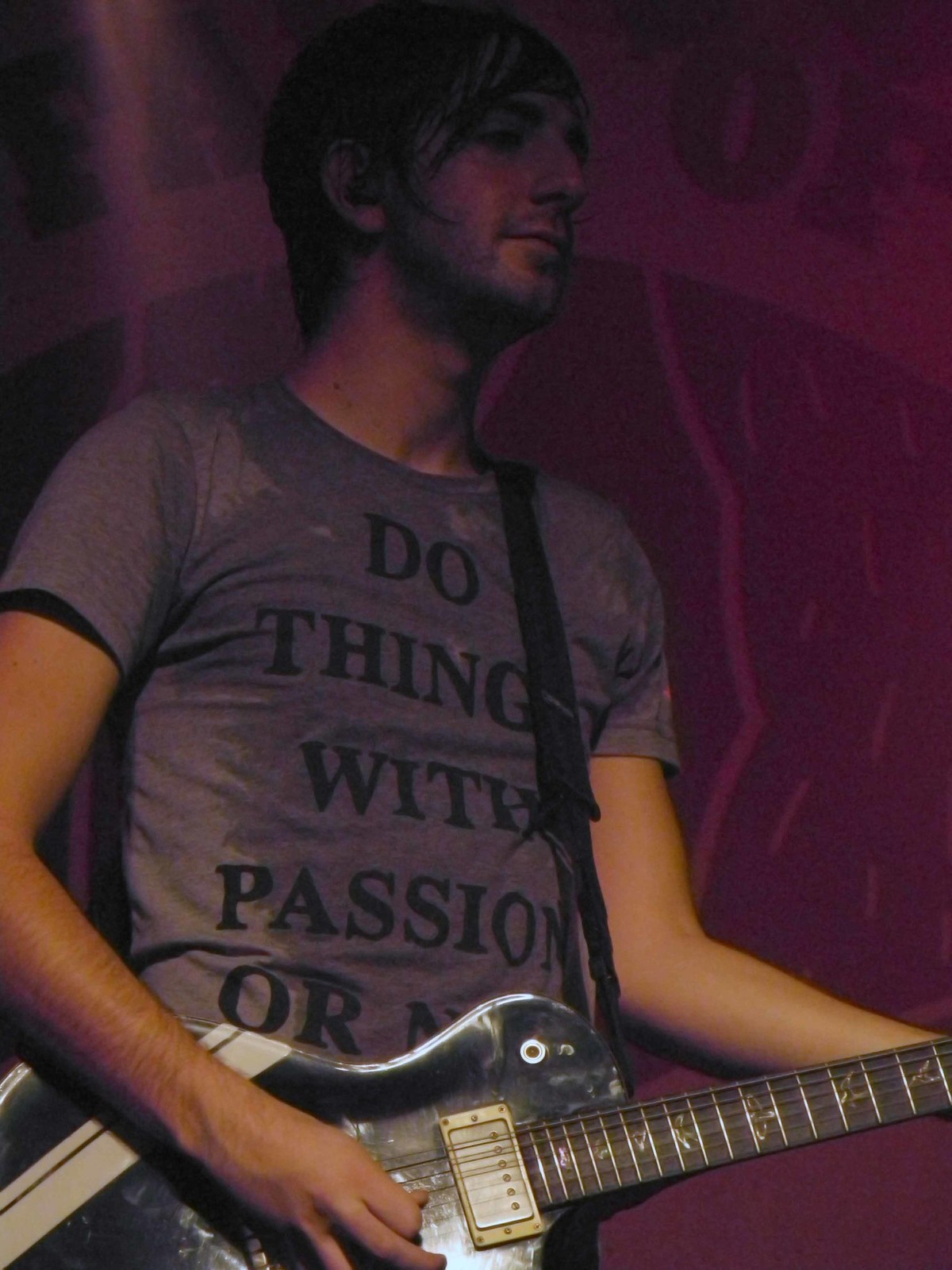This photograph captures a male guitarist deeply engrossed in his performance, set against a maroon background with an indistinct pattern. Sweat glistens on his face and soaks through his gray t-shirt, which features black lettering that partially reads "Do Things With Passion Or," with the remaining text obscured by the guitar. He has medium-length hair that clings to his forehead in sweaty bands, and a short beard. His electric guitar, black with white diagonal stripes and a brown neck, is slung over his left shoulder by a black strap. His left hand skillfully presses the strings while his right hand manipulates the chords. The lighting in the scene casts a purplish tint over the image, giving it a dynamic and moody ambiance. The guitarist's intense focus is directed off to the right, emphasizing his passion and immersion in the music.